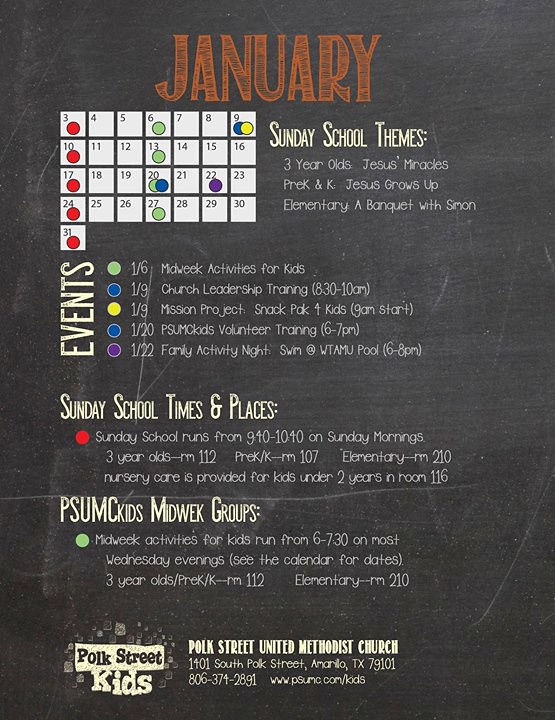The image is a detailed flyer from Polk Street United Methodist Church, featuring their Sunday school calendar for January. The background of the flyer is a dark blend of black and gray. At the top, the month "January" is prominently displayed in bold orange text. Below this, a calendar layout features white square boxes for each day, from the 3rd to the 31st, marked with colorful dots representing various events and activities. Red dots appear on all Sundays (3rd, 10th, 17th, 24th, and 31st), green dots on Wednesdays (6th, 13th, 20th, 27th), and additional blue, purple, and yellow dots scattered throughout.

To the right of the calendar, white text lists "Sunday School Themes" for different age groups: three-year-olds focus on "Jesus' Miracles," pre-kindergarten and kindergarten on "Jesus Grows Up," and elementary students on "A Banquet with Simon." Below the calendar, event details are provided in a vertical format, explaining the significance of the dots: green for mid-week activities for kids, blue for church leadership training, yellow for mission projects, another blue for PSUMC kids volunteer training, and purple for family activity night events.

Further down, bold text outlines Sunday school times and places, noting classes for three-year-olds and pre-K to kindergarten in specific rooms, and elementary classes in another. Nursery care for kids under two is indicated in room 116. Another section details mid-week groups for kids, running from 6:00 to 7:30 PM on most Wednesday evenings, specifying rooms for different age groups.

At the bottom left, the Polk Street Kids logo is visible next to the church's full name, address at 1401 South Polk Street, Amarillo, TX 79101, and contact information including phone number and website (www.psumc.com/kids).